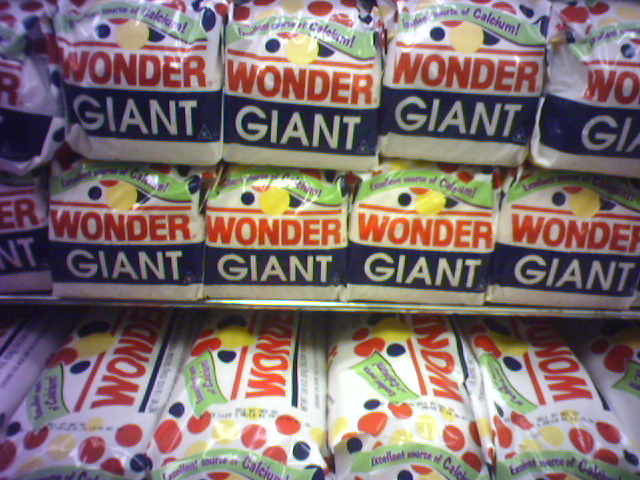This color photograph captures a neatly organized display of Wonder Bread at a grocery store. The image focuses on several wire shelves loaded with rows of Wonder Giant Bread. The top shelf features two stacks of six loaves each, all aligned with the bottom ends facing the camera, while the bottom shelf holds about six loaves in a similar arrangement. Each loaf is wrapped in the iconic white Wonder Bread packaging, which prominently features the brand name "Wonder" in bold red letters, accompanied by a blue banner that reads "Giant" in contrasting white text. The packaging is adorned with the brand's signature colorful polka dots—red, blue, and yellow—adding a vibrant touch to the uniform display of bread. The ties on the packaging are not visible, emphasizing the consistent orientation of the loaves.